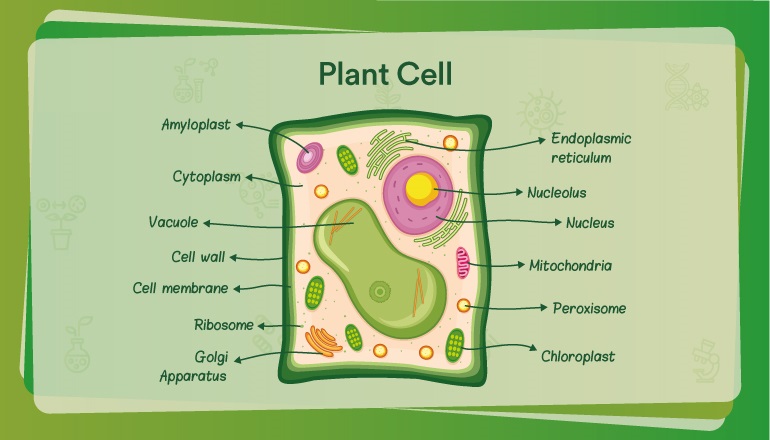This illustration is a three-dimensional, animated depiction of a plant cell, likely sourced from a high school textbook. The rectangular image is bordered with a bright green frame, and the interior background is a light mint green. Within this background, various substructures of the plant cell are meticulously labeled with green text and arrows pointing to each component. Key labeled components include the endoplasmic reticulum, nucleolus, nucleus, mitochondria, peroxisome, chloroplast, Golgi apparatus, ribosome, cell membrane, cell wall, vacuole, cytoplasm, and amyloplast.

The cell wall is depicted as a square, enclosing all the internal elements of the plant cell. These components are color-coded in shades of light purple, light green, light yellow, and other colors such as orange and pink to differentiate them. Additionally, the green background features smaller illustrations in varied green shades, showing a microscope, an animated virus cell, and a vase with flowers, further enhancing the educational aspect of the image. This descriptive and colorful layout emphasizes the key structures and their roles within the plant cell, making it a detailed and comprehensive visual aid for learning.